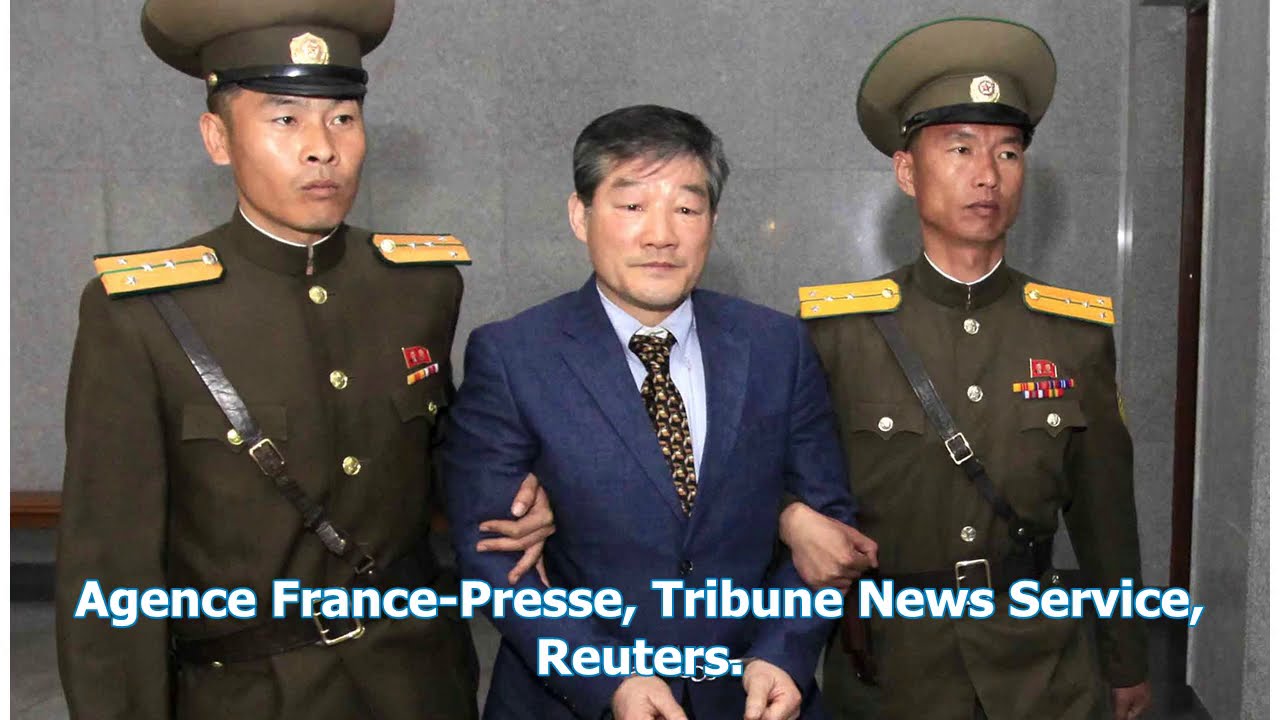In the photograph, a middle-aged Asian man in a navy blue suit, white shirt, and multicolored tie is being led away in handcuffs by two stern-looking Asian men in highly stylized brown military uniforms. The detained man, appearing to be in his 40s or 50s, is flanked by the two officers, each with large green hats adorned with gold badges, gold epaulets on their shoulders, and dark belts with black sashes across their chests. The uniforms feature gold buttons and medals on the left chest, making them look official and imposing. Both officers have looped their arms through those of the handcuffed man, firmly holding him as they walk in front of a gray wall, possibly suggesting a courthouse or similar somber setting. In white text at the bottom of the image, the photograph is credited to Agence France-Presse, Tribune News Service, and Reuters. The atmosphere is grave, with all men displaying serious expressions.